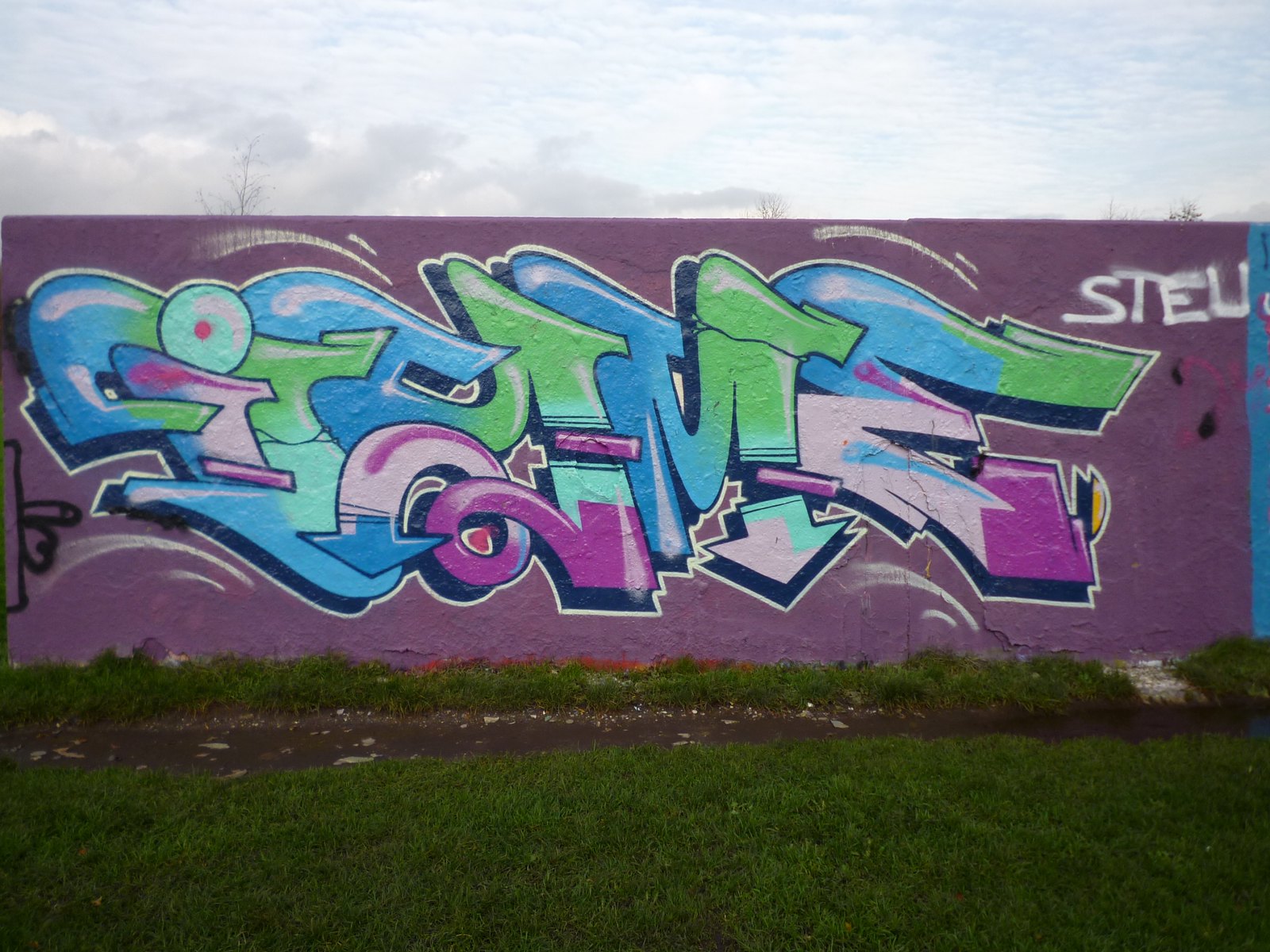The image depicts an outdoor scene with a prominent concrete wall painted in a darker gray-purple hue, adorned with vibrant graffiti art. The graffiti features wild and large letters that appear to spell out "slime," though the elaborate style, including arrow-like ends on some letters, makes it challenging to decipher. The lettering showcases a mix of light pink, purple, baby blue, and lime green, with some letters fading from blue into green. Additionally, the upper right corner of the wall distinctly displays the letters "STU" in a more readable form. In the foreground, there is dark green grass, followed by a weathered pathway dotted with asphalt, dirt, litter, and branches. Another patch of rough grass borders this path. Above the wall, the backdrop includes a sky with wispy white clouds and a few tree branches peeking in from the left, creating a picturesque yet urban setting.